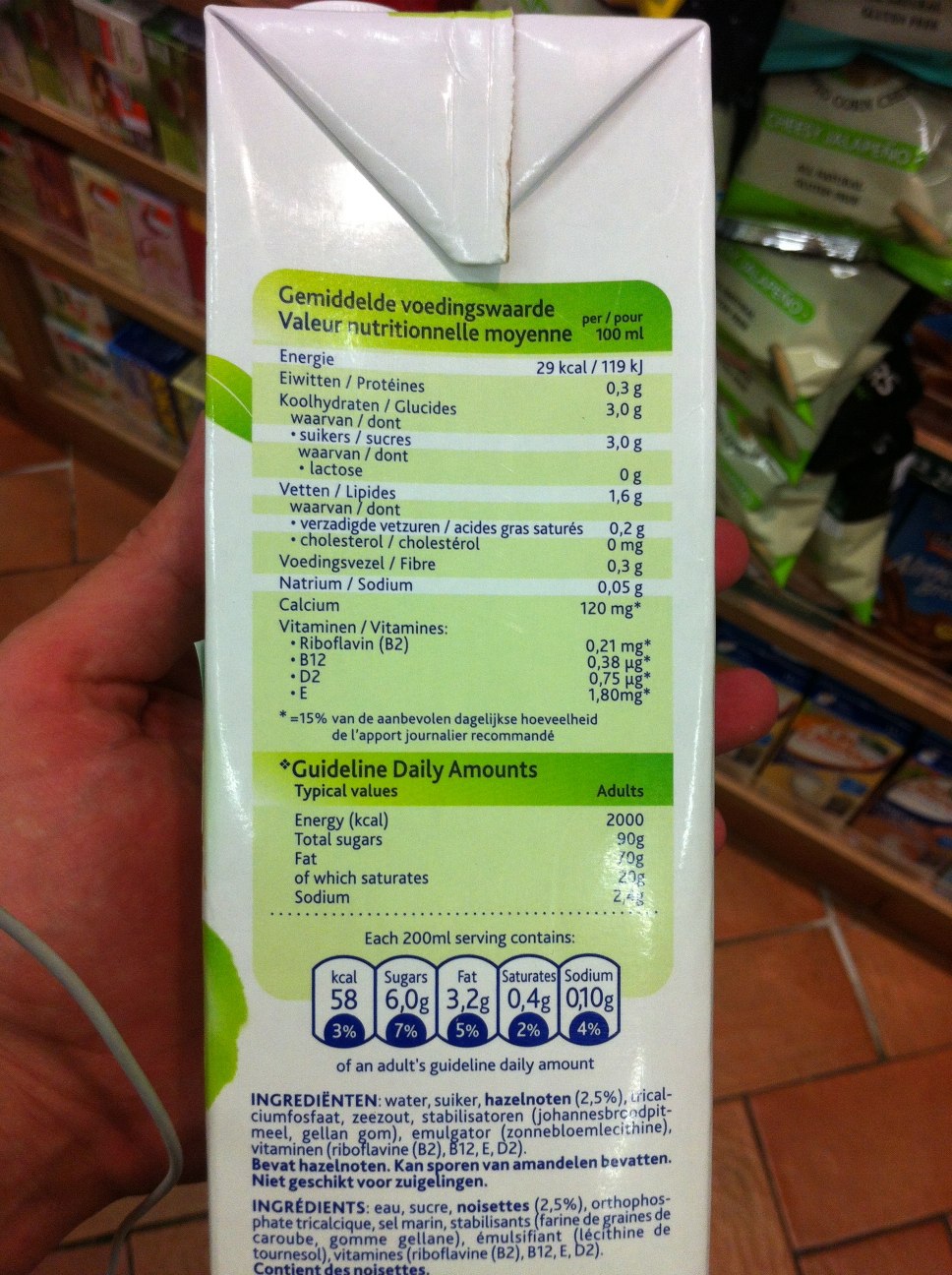In this vertically oriented rectangular image, a hand emerges from the lower left corner holding a drink carton. The carton, predominantly white, features a small twist-off cap on top and a folded triangular section at its peak. The side of the carton displays nutritional information against a green background with white stripes. The text, seemingly in a foreign language, reads: "Gemidaldi Voding Suard, Valure Nutritionnelle Moyenne, Energy 29 Kcal, Proteins 0.3g, Glucides 3g, Lipides 1.6g, Sodium 0.5g." Below, guidelines suggest daily amounts for typical adults: "Energy 2000 Kcal, Total Sugars 90g, Fat (illegible), Saturates 20g, Sodium 2 (illegible digits)." Further nutritional values listed are: 58 Kcals, 6g Sugar, 3.2g Fat, 0.4g Saturates, and 0.10g Sodium.